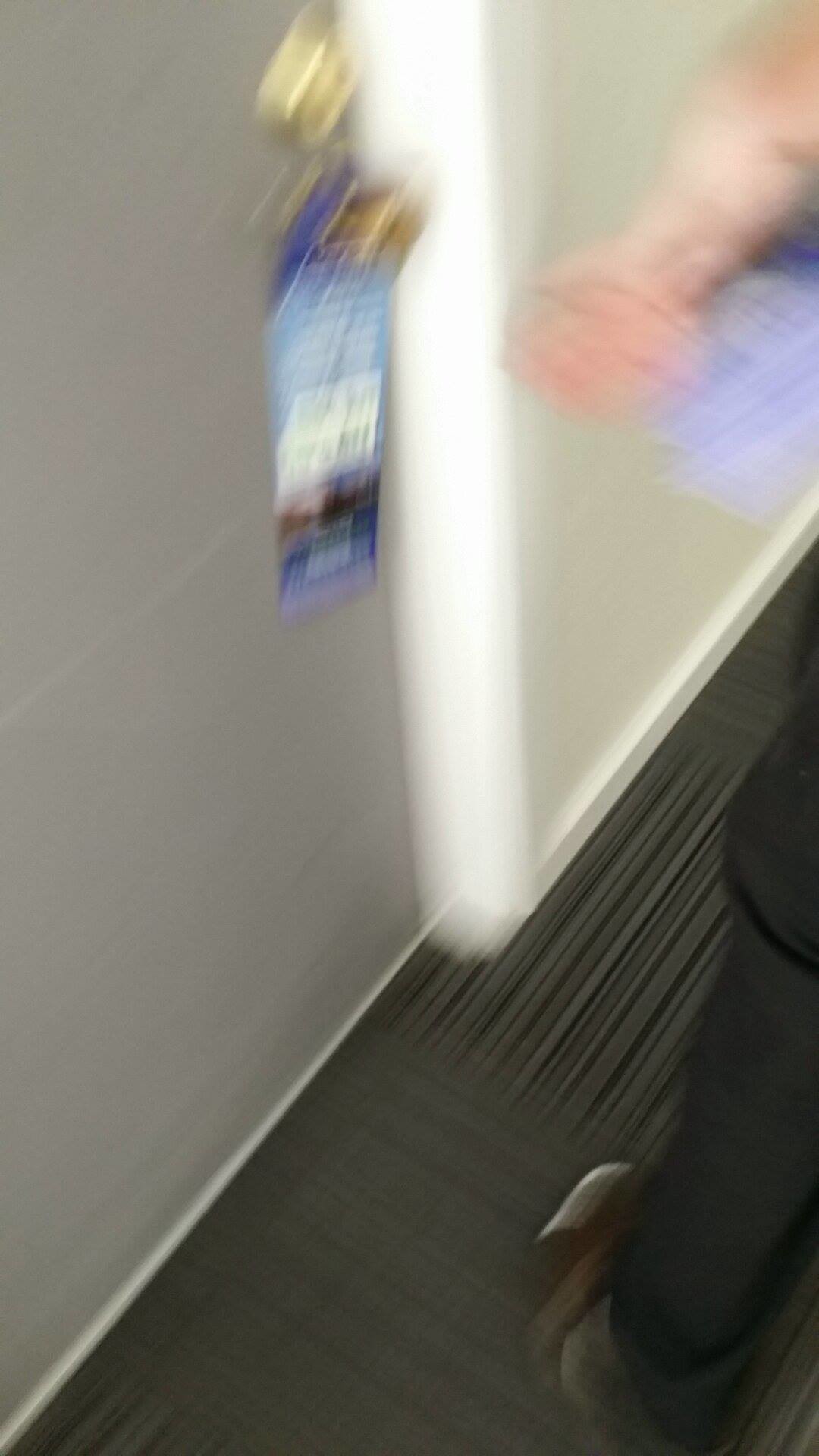The image depicts a blurry hallway likely in a hotel, characterized by industrial-style gray and black striped carpet tiles on the floor. The hallway has white walls and a white door with a brass or gold handle. A bolt lock is visible on the door, adding to the security detail. Hanging on the handle is a blue and white sign, typically resembling a "Do Not Disturb" notice, but its text is illegible due to the blur. The sign seems to feature a picture of a maid's uniform with an outstretched hand. In the image, there appears to be a person with light skin tone, wearing black pants and possibly brown shoes, holding a blue item—potentially similar to the signs on the door—as they move, indicating motion blur in the photo.